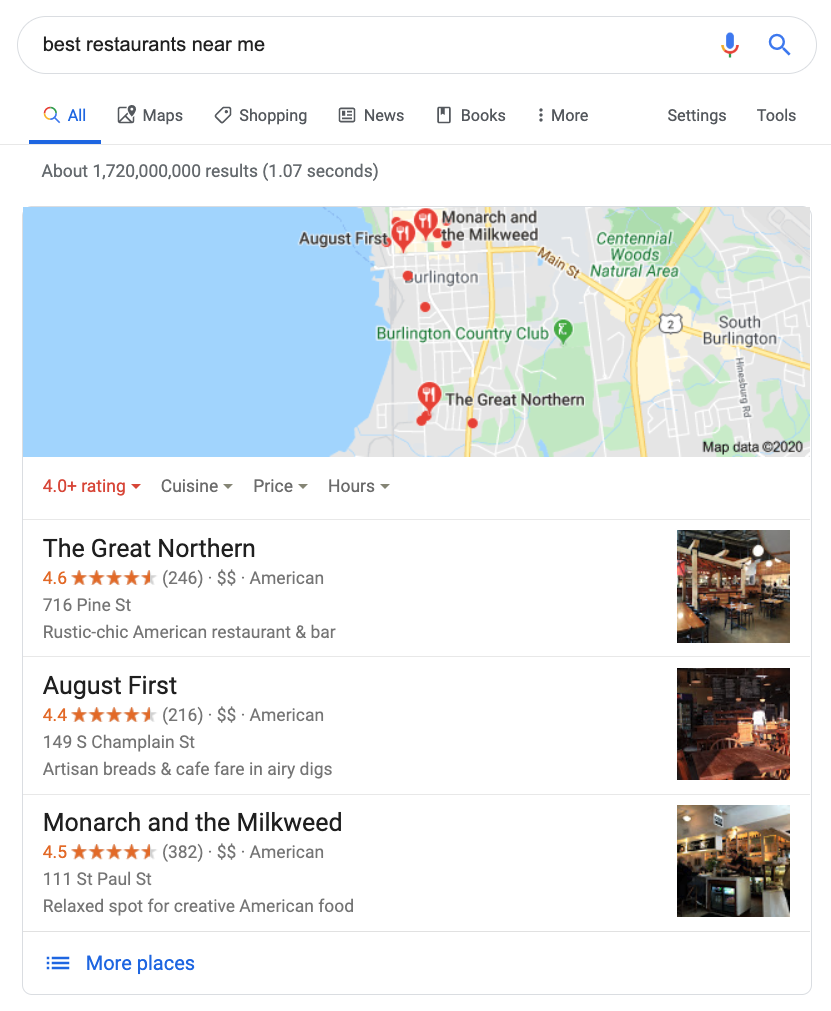The image showcases a Google Maps page on a website, illustrating a search for the best nearby restaurants. At the top, the familiar Google search box is visible, with various tabs including All, Maps, Shopping, News, Books, More, Settings, and Tools, clearly indicating that the user has selected the "All" tab. Below the search bar is a dynamic map displaying several results, each marked with pinpoint icons.

Accompanying the map is a side panel listing the top-rated dining options, each with detailed ratings and relevant information. Highlighted in this panel are:

1. **The Great Northern** - boasting a stellar rating of 4.6 stars.
2. **August 1st** - which has garnered a commendable 4.4 stars.
3. **Monarch and the Milkweed** - achieving a solid rating of 4.5 stars.

Additionally, the interface includes options for filtering results by gasoline prices and operating hours, ensuring a comprehensive exploratory experience. Below these top listings, there is an option to view "More places."